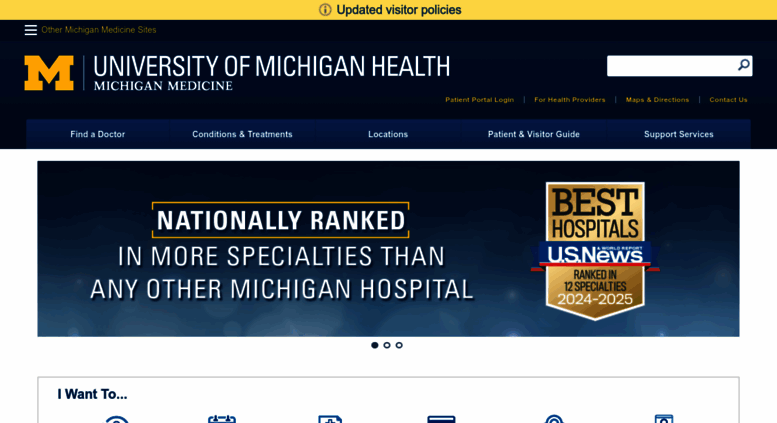**Descriptive Caption:**

Screenshot of the University of Michigan Health, Michigan Medical Center Homepage

This image showcases the homepage of the University of Michigan Health, Michigan Medical Center website, designed primarily for individuals seeking medical information or looking to find a doctor. As the dominant school color, blue is prominently featured throughout the site, accented by the university's signature maize (gold) color.

At the top of the webpage, a noticeable yellow banner presents updated visitor policies. Below the banner, the University of Michigan Health logo is visible alongside a functional search bar and quick-access links such as patient portal login, health provider resources, maps and directions, and a contact us option.

Further down, the navigation menu categories are clearly labeled: Find a Doctor, Conditions & Treatments, Locations, Patient & Visitor Guide, and Support Services, offering streamlined navigation for users. Another visual feature includes a congratulatory banner celebrating Michigan as the number one hospital, alongside the Best Hospitals US News logo for the 2023 to 2024 period.

Just beneath this, partially visible logos provide access to various options indicated by an "I want to" prompt, with actionable icons slightly cut off in the screenshot. The overall website layout appears user-friendly, combining a predominantly blue palette with white accents for clarity and ease of use.